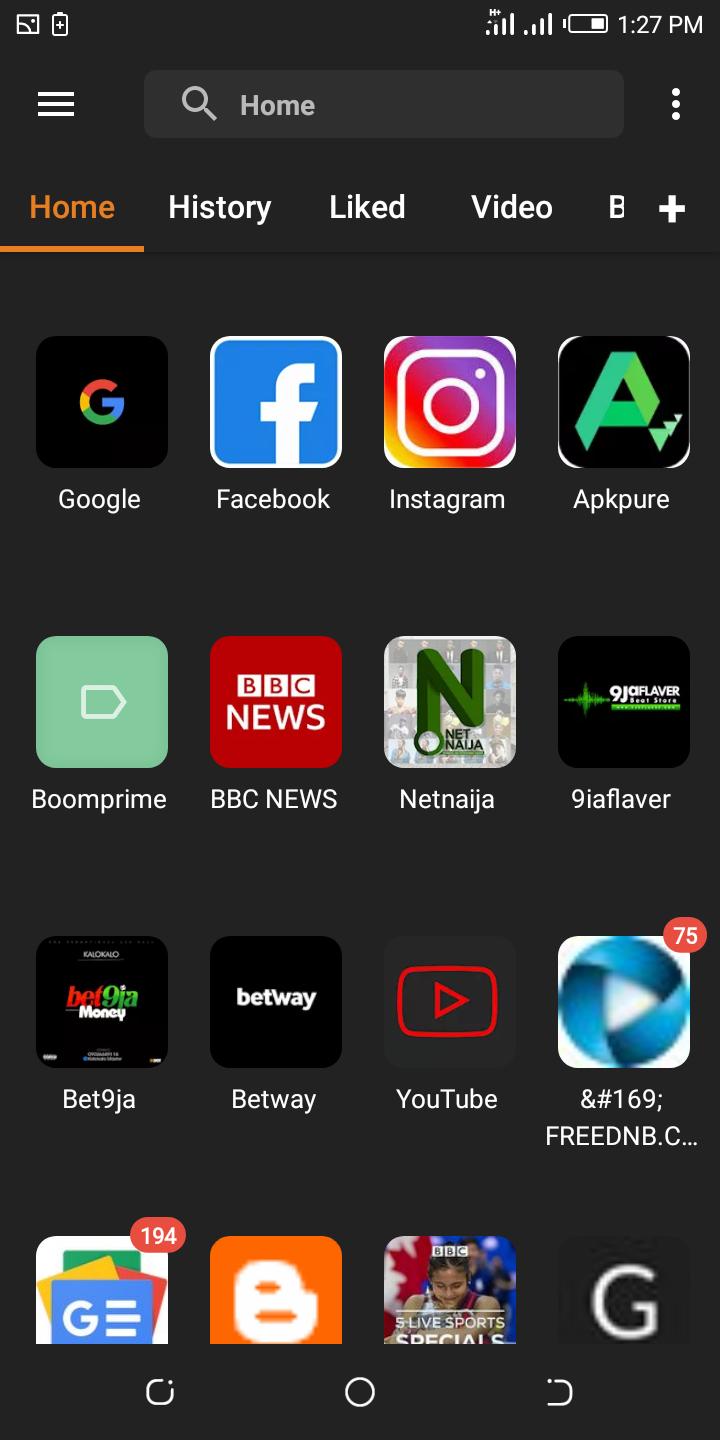Screenshot of a mobile phone's home screen taken at 1:27 PM. The phone is in portrait mode with battery-saving mode enabled, displaying approximately two-thirds battery remaining. Full Wi-Fi bars are visible, connected to two different networks. The top section features a home search bar, with the Home menu currently selected and highlighted in orange. Adjacent tabs include History, Liked Videos, and a 'B+' option indicating more scrollable content.

Apps installed on the home screen are as follows:
1. **Google** - Represented by the Google logo.
2. **Facebook** - Icon with a white 'f' on a blue background.
3. **Instagram** - Recognizable by its rainbow-colored camera icon.
4. **Aka KP Pure** - An application installer bypassing the Google Play Store.
5. **Boom Prime** - Displayed with a house-shaped triangle icon.
6. **BBC News** - Red background with white lettering.
7. **Net Analogy** - Illustrated by a large green 'N.'
8. **Nine IA Flavor** - Appears to be a sound editing program.
9. **Bet Ninja and Bet Away** - Likely gambling applications.
10. **YouTube** - Classic red play button icon.
11. **Free DBNC** - Has accompanying notifications.
12. **Google Cluster** - Listing 194 warnings.

The bottom navigation bar includes icons for Home, Context Menu, and Back, along with live sports special access from BBC and Google.